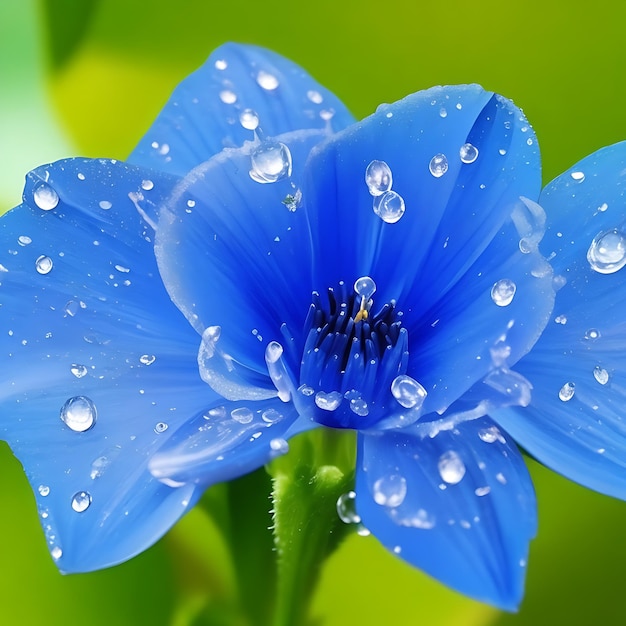This striking macro photograph captures a hyper-realistic, vibrant blue flower adorned with crystal-clear raindrops. The flower appears almost surreal with its sharply detailed petals and ethereal quality. The petals gradient from a purplish dark blue at the center to a lighter blue at the edges, creating a mesmerizing transition of hues. It features a rosette-like center resembling a crown, composed of multiple petals and prominently displaying a yellow stamen surrounded by the intricate arrangement. The photograph’s precise focus highlights the water droplets, varying in size, that cling to the petals, enhancing their brilliance and texture. The background, though blurred and green, complements the vivid blue and creates a natural frame around the flower, accentuating its color and minute details. The entire composition, set against an out-of-focus green stem and surrounding foliage, intensifies the flower's stunning beauty, making it seem more like an artwork than a mere photograph.